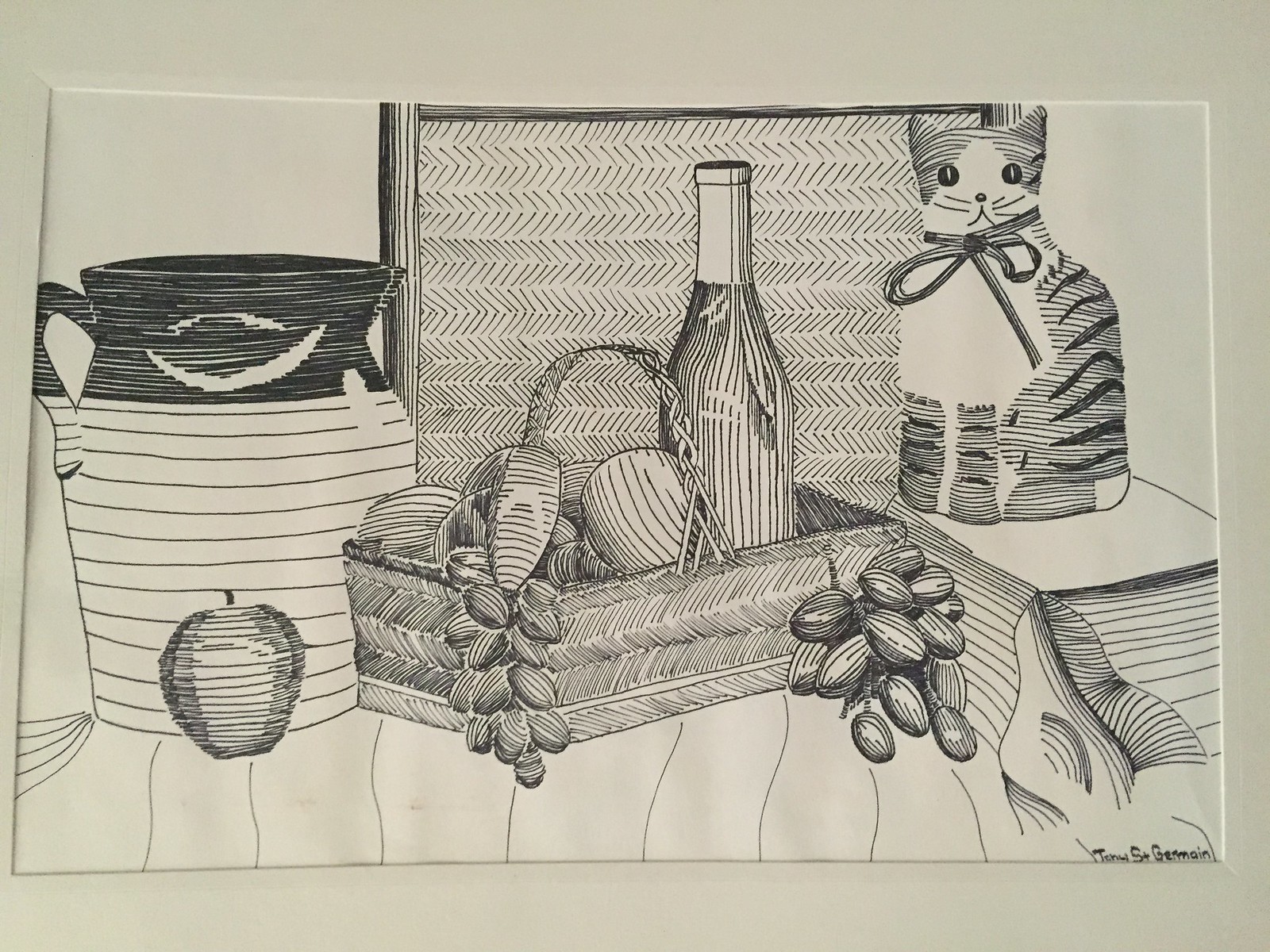This detailed black pen sketch, rendered on a sheet of white paper and set against a matching white surface, captures an intricate still life scene. Central to the composition is a rectangular basket filled with fruit, including bunches of grapes spilling over the sides. Nestled among the fruit is a bottle of wine, adding a touch of elegance to the arrangement. To the left of the basket, an apple and a jug with a black top and delicate leaf detail are meticulously depicted, further enriching the scene. The tabletop they rest on is adorned with stripes, adding texture and depth. In the background, a small stack (possibly books or a stand) supports a charming cat figurine, while a framed, cross-hatched image provides a subtle yet striking backdrop. The artwork is discreetly signed in the lower right-hand corner, though the signature is somewhat difficult to decipher, seemingly reading "To New St. Germain." This detailed composition beautifully showcases the artist's skill in capturing everyday objects with precision and artistic flair.